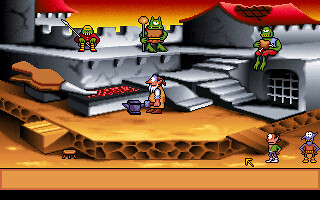In this video game level, the scene unfolds with a layered background, starting at the bottom with a horizontal black strip, giving way to a light orangish-brown backdrop. This serves as the foundation for the level itself. At the forefront, two characters stand out: a blue goblin and a person clad in green attire. A small yellow arrow points upward, guiding players' attention to the gameplay elements.

The level design features several ramps that ascend to an upper platform. The edge of this platform is brown and marked by noticeable holes, while the main flooring is a lighter shade of brown. Among the characters, a side view reveals an elderly figure with a white beard, dressed in brown and holding a distinctive purple watering can.

To the right of the scene, gray stairs ascend to the highest platform level, where three green, alien-like characters are either resting or standing. Two housing structures with red roofs are placed in the upper right and left corners of the image. The background sky at the top adds a colorful touch with its gradient of yellow and red hues. This detailed tableau combines various elements to create an engaging and visually rich game level.